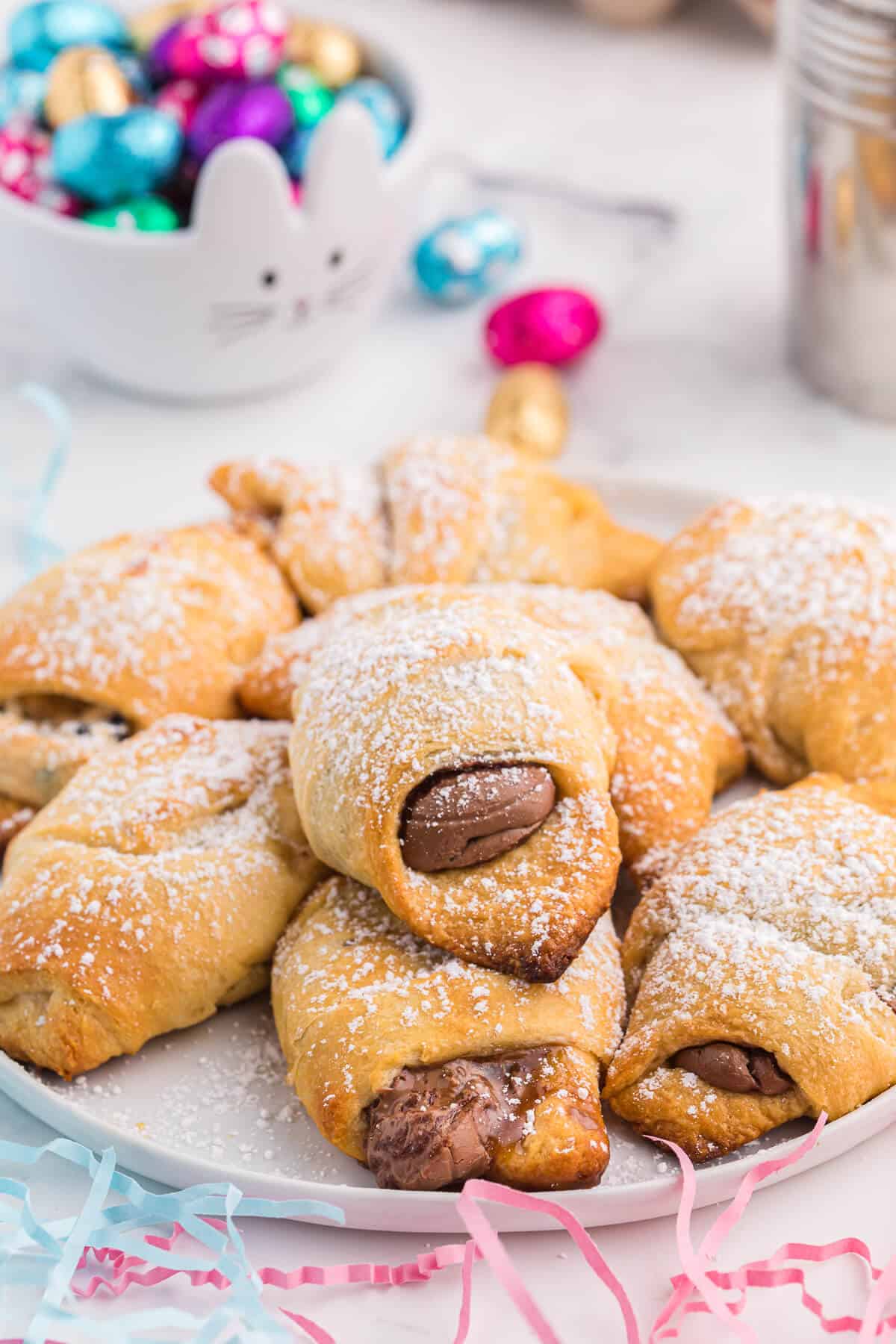The image is a detailed indoor photograph featuring a dessert setting. At the center is a white round plate positioned on a white tablecloth adorned with blue and pink confetti or streamers. The plate holds a pile of buttery, browned croissant-like pastries filled with a chocolate custard and generously dusted with powdered sugar. In the background, slightly blurred, is a white plastic bowl shaped like an Easter bunny head, complete with raised ears, black eyes, a pink nose, and whiskers. This bowl is filled with colorful, foil-wrapped chocolate eggs, with some eggs scattered outside around the bowl. The foils come in an array of colors, including blue, pink, purple, and gold. To the upper right of the scene sits some sort of a silver cup, adding an additional metallic contrast to the festive arrangement.